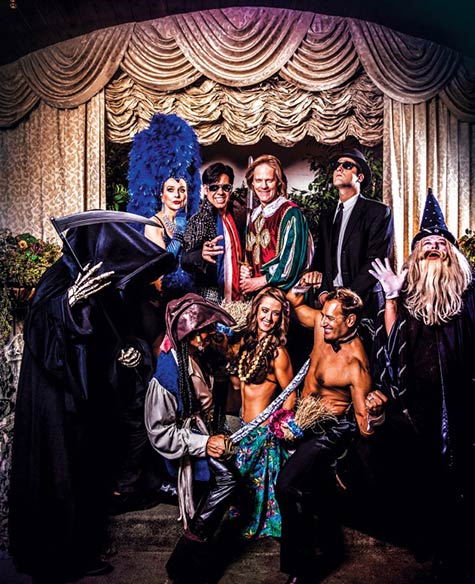The image appears to be an elaborate, vibrant poster for a theatrical production, possibly from the 1950s or 60s, featuring a diverse cast of characters in elaborate costumes. The backdrop is a richly designed theatrical curtain, adding to the drama and intricacy of the scene. To the left, a figure dressed as the Grim Reaper looms, complete with a dark cloak and skeleton hands. At the center, attention is drawn to a woman adorned in a bright blue feathered headdress, resembling a Vegas showgirl, flanked by a man who seems to be dressed as Elvis Presley or a rock star. To her side, another man stands, looking like a detective or agent with sunglasses and a hat. Adding to the eclectic mix, a wizard, complete with a wizard's hat, stands to the right, while a man dressed in regal or aristocratic attire adds a touch of royalty. Below this main group, at center stage, a shirtless man who resembles a Chip and Dale dancer smiles beside a woman in a bikini and sarong, evoking a Hawaiian theme. Nearby, a playful pirate aims his sword at the dancer, adding a hint of mischief. The entire ensemble suggests a lively, Halloween-like photoshoot or a promotional poster for a Broadway play, capturing the essence of different characters and styles from various genres.